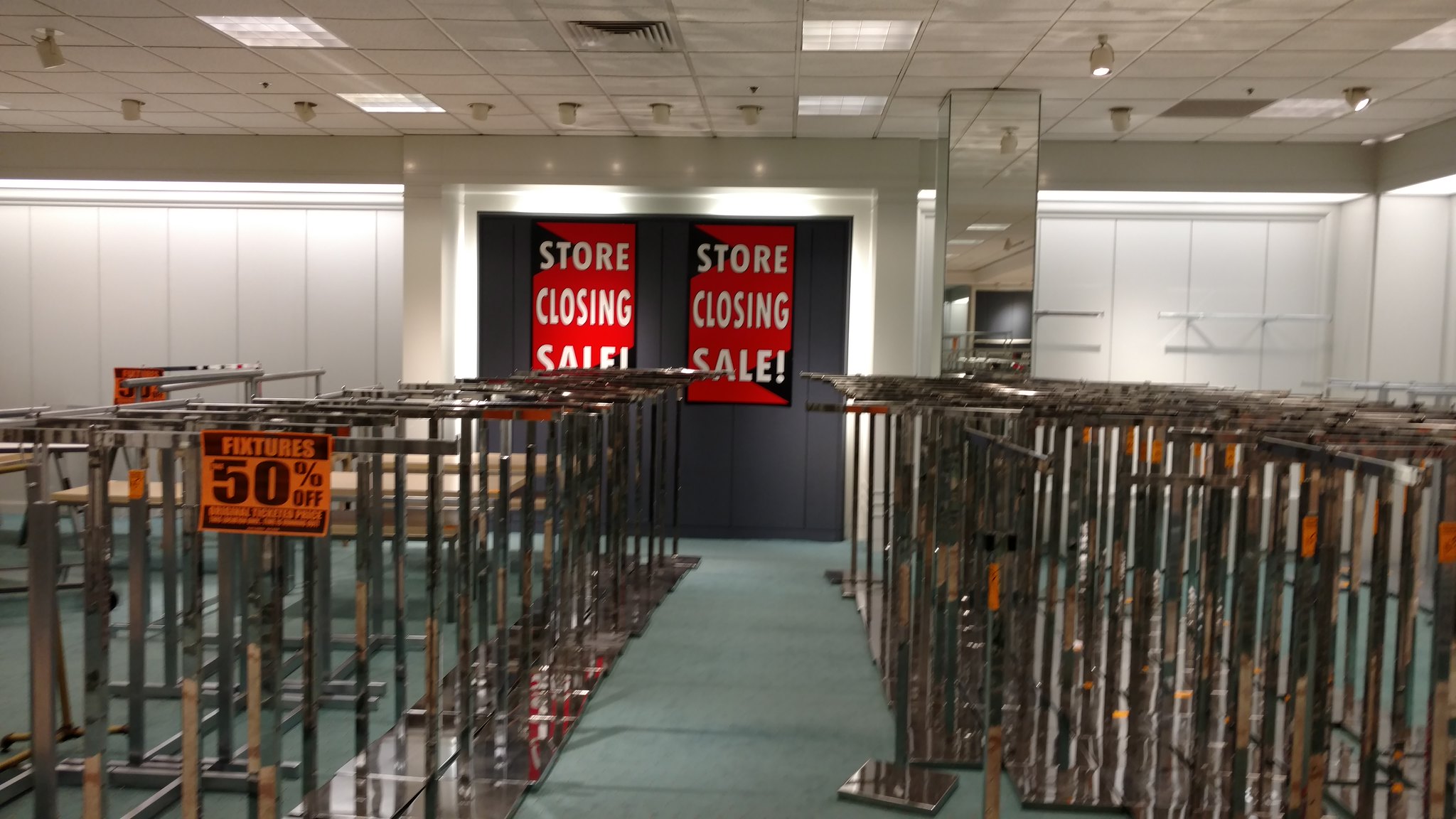The image depicts the interior of an empty department store, primarily focused on the blue-floored area lined with multiple brown cages, which were probably used for displaying merchandise. The store appears to be in the process of liquidating, evidenced by an orange sign in the front left cage that reads "Fixtures 50% Off," and two prominent signs against the black section of the far wall that declare "Store Closing Sale" in white text on a red background. The store is well-lit with ceiling lights, revealing the white walls flanking both sides of the space. A pillar on the right side with mirrored surfaces adds to the scene of an abandoned retail environment where even the display items are up for sale.